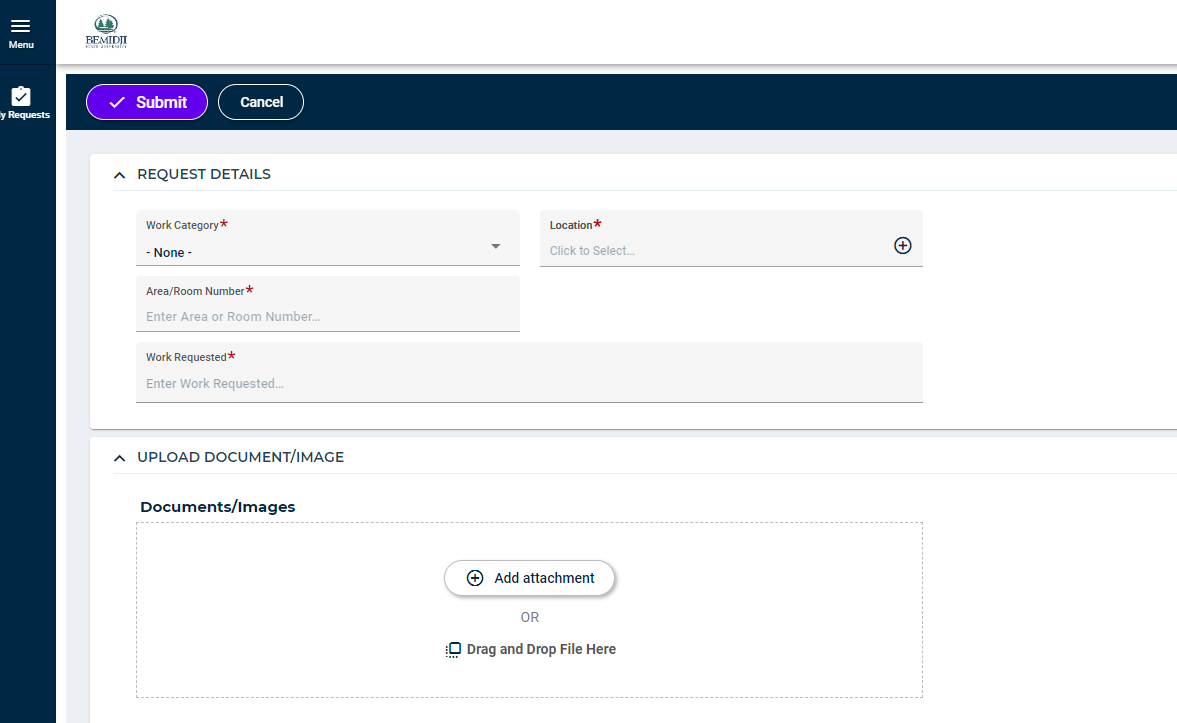The website depicted in the image is titled "Bemidji" (spelled B-E-M-I-D-J-I). The resolution of the image is poor, making it difficult to read the text directly below the title. The webpage has a dark blue vertical navigation bar on the left side. At the top left corner of this bar, there's an icon with the word "Menu" above three horizontal lines, followed by the word "Requests" beside an icon of a clipboard with a checkmark.

To the right of the title "Bemidji", there is a thin blue horizontal line that spans across the screen. Below this line, there is a purple "Submit" button on the left and a grey "Cancel" button on the right.

Underneath these buttons, the page features several form fields labeled with red asterisks to indicate mandatory input. The fields are:
1. **Work Company** – Displays a dropdown menu labeled "None."
2. **Area/Room Number** – An input field labeled "Enter area or room number."
3. **Work Requested** – A blank input field for entering a work request.
4. **Location** – An interactive field labeled "Click to select location," with a circle containing a plus sign on the far right.

Below the form fields, there is an option to upload documents or images, titled "Upload Document/Image," with the subtext "Add attachments or drag and drop files here."

The background of the webpage is predominantly white, providing a clean and simple interface.